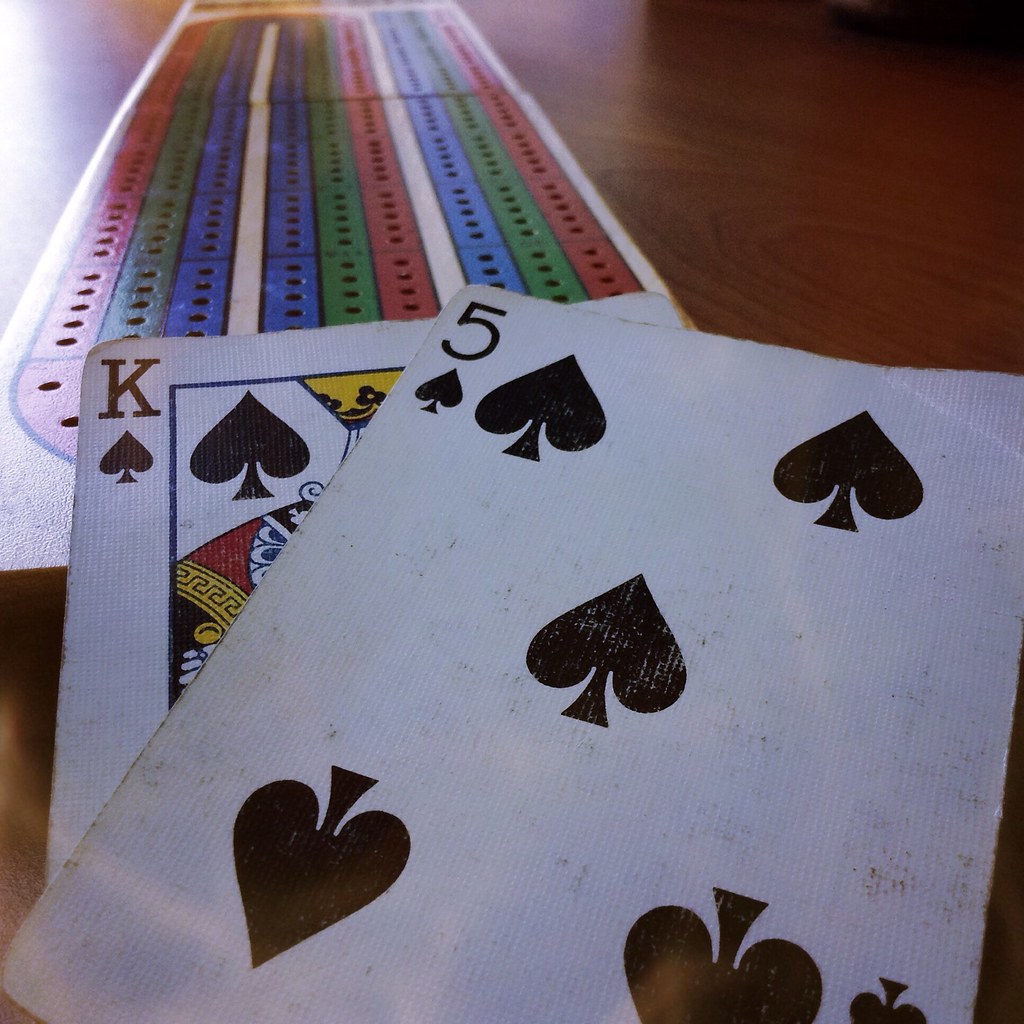A polished brown table is adorned with a dazzling finish, reflecting the light from an open window and a door on the opposite side. Prominently placed on the table are two playing cards, a five of spades and a king of spades. Stretching out along the table is an elongated white board showcasing an intricate pattern of vibrant stripes in a sequence of red, green, blue, and white, repeating multiple times. Towards the rounded end of the board, the specific color is not discernible, but the colorful pattern continues in a cohesive manner. This board, possibly part of a game, features numerous peg holes, each holding small brick-like pieces with four holes in a systematic arrangement, stacked end to end along various lines.